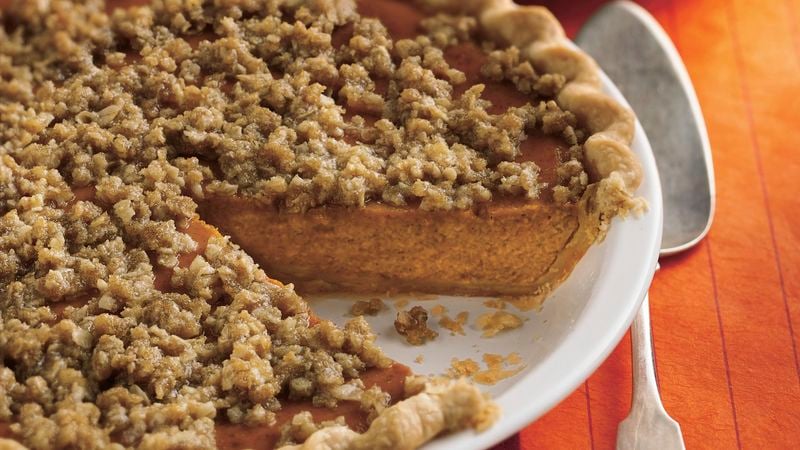This detailed, color photograph captures a close-up of a pumpkin pie with a streusel topping, set in a white ceramic pie dish. The image, taken in landscape orientation, shows the pie positioned nearly centered but slightly offset to the right. A single slice of the pie is missing, revealing the creamy orange filling and the thickness of the crimped, golden crust. The streusel topping is a light brown color, adding texture to the smooth surface of the pie. Adjacent to the pie dish is a silver pie server, laying vertically against the right edge of the dish on an orange napkin accentuated with dark stripes. Both the pie and server rest upon a tabletop made of reddish-colored wood planks, lit naturally to emphasize the clarity and details of the photograph. The overall composition resonates with a warm, inviting atmosphere, typical of high-quality food photography.